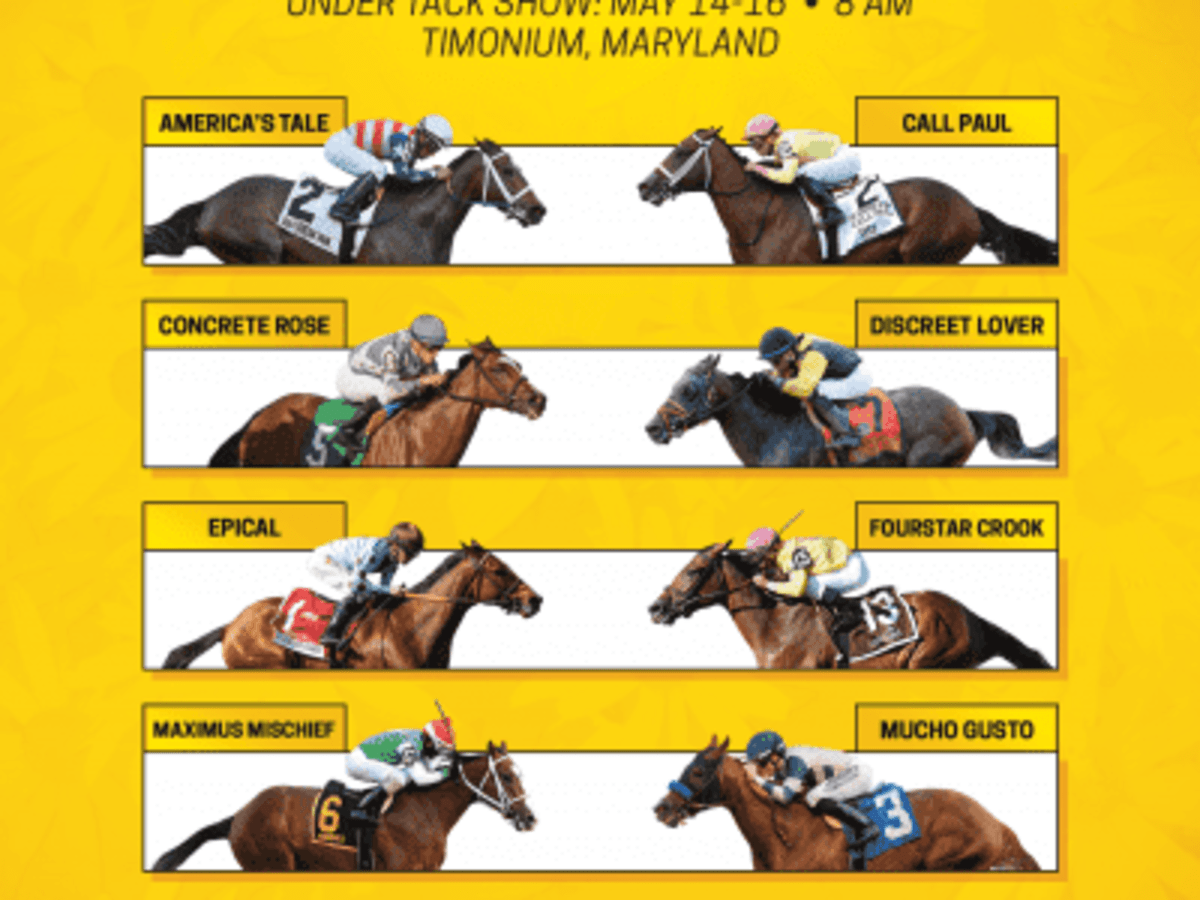The image is a promotional poster for an Under Tack Show, scheduled for May 14-16 at 8 a.m., located in Timonium, Maryland. Set against a mustard-yellow background, the poster features four white horizontal rectangles, each displaying two horses with their jockeys in colorful racing gear. Each pair of horses faces each other, with names listed above them. 

In the first row, "America's Tale" is on the left and "Call Paul" is on the right. The second row features "Concrete Rose" on the left and "Discreet Lover" on the right. The third row shows "Epical" on the left and "Four Star Crook" on the right. Finally, the bottom row includes "Maximus Mischief" on the left and "Mucho Gusto" on the right. The jockeys wear distinctive outfits and number decals, hinting at an upcoming race.